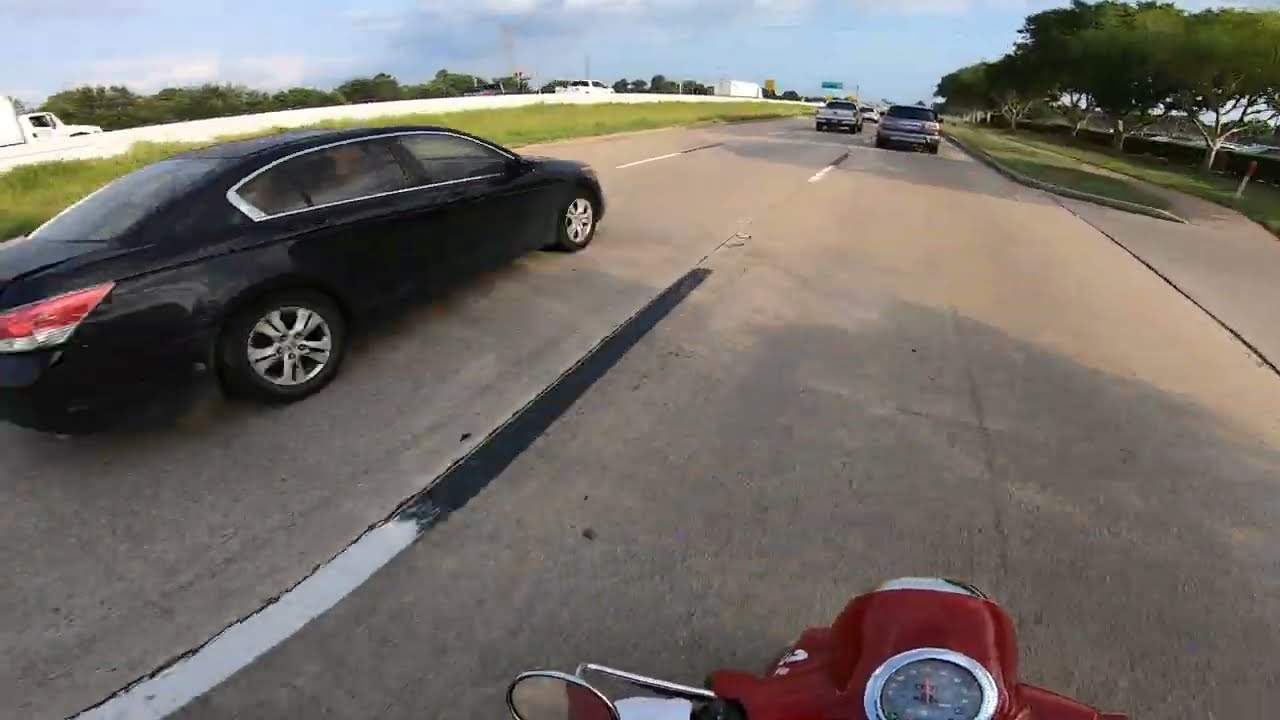A vibrant photograph taken from the perspective of a motorcycle rider, possibly equipped with a dash cam, on an expansive six-lane highway. The well-paved road features distinct white and black lane markings against its gray surface. At the bottom of the image, the motorcycle's red body and chrome accents are prominently displayed, including a speedometer with a black background and white lettering. 

In the adjacent left lane, there is a black sedan slightly ahead of the motorcycle. Directly in front of the motorcycle is a silver vehicle, which appears to be an SUV, joined further ahead by a white pickup truck. To the right side of the highway, thick green vegetation and trees line the road, contrasting with the blue sky and scattered clouds above.

On the opposite side of the highway, separated by a divider strip filled with grass and bushes, is another set of lanes with sparse traffic, including at least two white vehicles. The scene confidently suggests a pleasant day with clear visibility, enhancing the overall impression of a leisurely ride amid verdant surroundings and open sky.